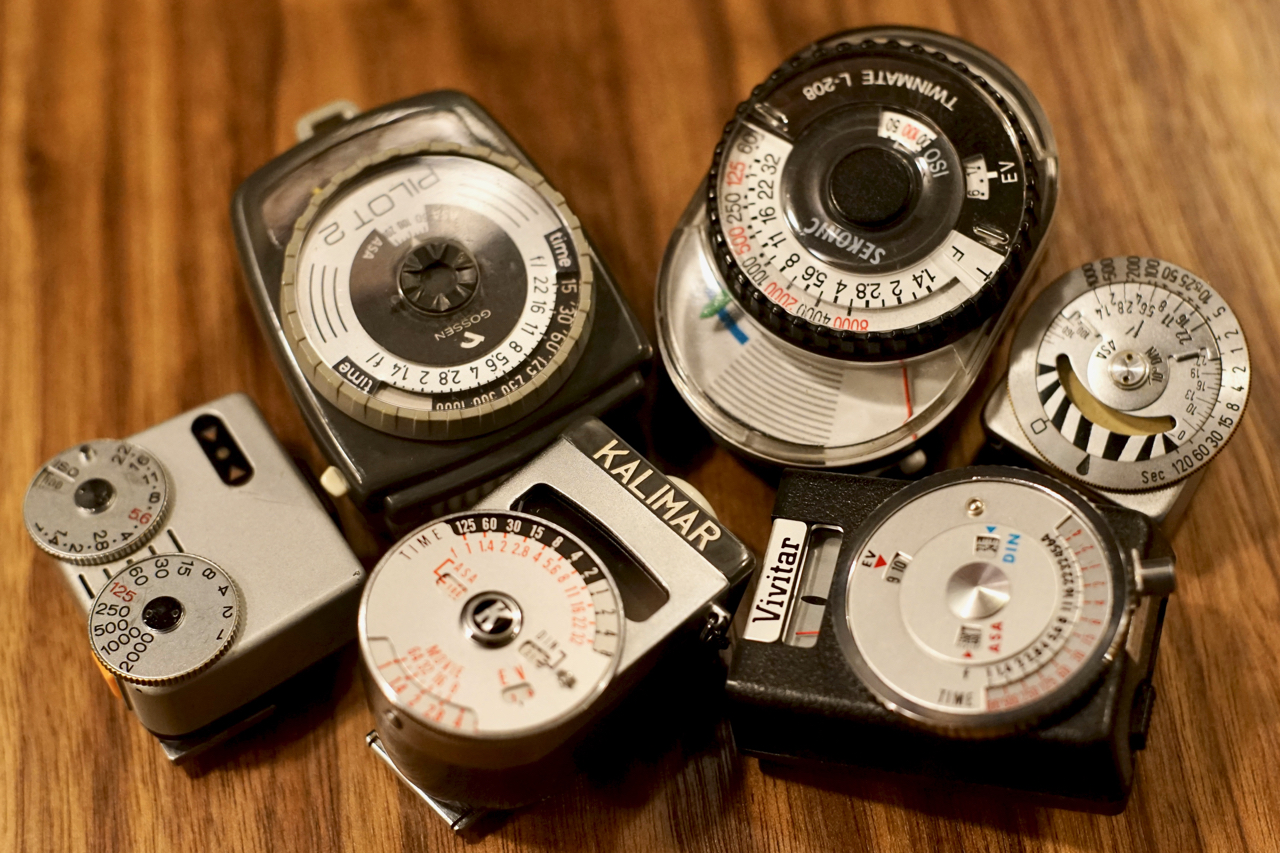The image depicts six small, vintage-looking devices identified as light meters, meticulously arranged on a wooden table. Each light meter showcases its intricate dials and gauges, designed to measure light exposure. The devices, mostly cylindrical and fitting comfortably in the palm of a hand, are branded with various names: Pilot II, Sekonic, Vivitar, Calimar, and Gossen Pilot II. Notably, the far-left and far-right meters lack visible branding, with the far-left device distinguished by its unique configuration of two small dials, contrasting with the larger, round dials on the others. The detailed craftsmanship and variety in the dials hint at their specialized use in photography, capturing different aspects of light measurement.